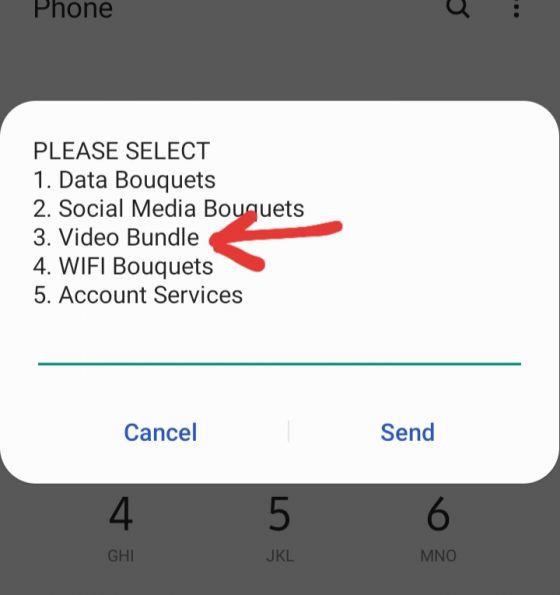The image showcases a smartphone interface with a semi-transparent background displaying a typical phone keypad. In the upper left corner of the background, the word "Phone" appears in black font. On the upper right corner, there are two icons: a magnifying glass for search and a vertical ellipsis representing additional options.

Dominating the screen is a white, rounded-corner pop-up window that occupies the majority of the image. This pop-up extends fully to the right side and off the left side of the image, resulting in a partially cut-off view on the left. The pop-up window presents a list titled "Please select," followed by five options:

1. Data Bouquets
2. Social Media Bouquets
3. Video Bundle (highlighted with a red arrow pointing to it)
4. Wi-Fi Bouquets
5. Account Services